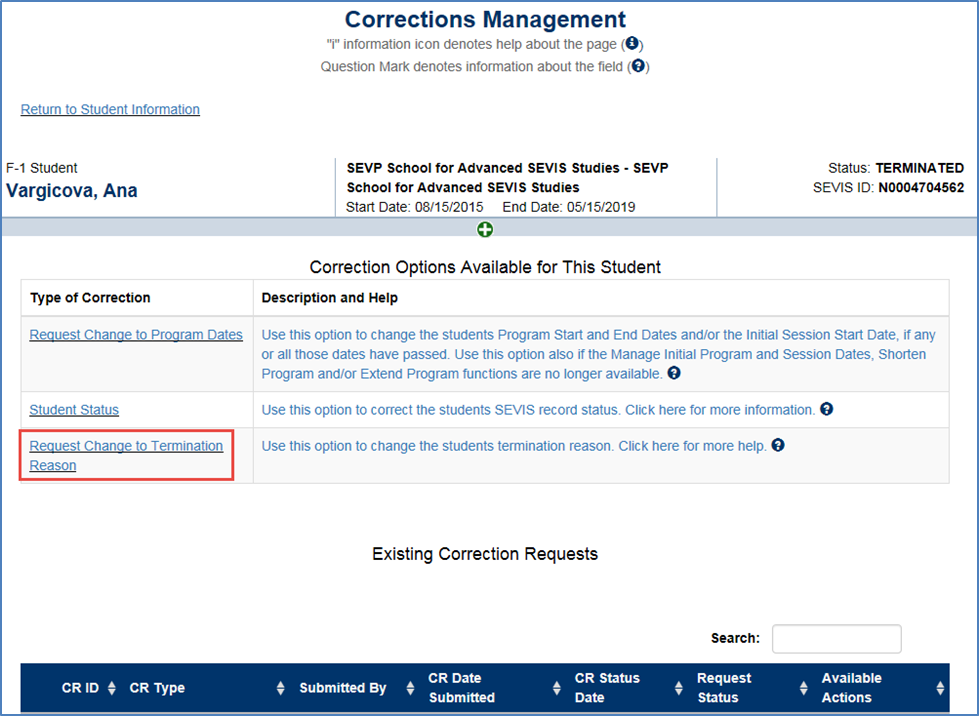The screenshot captures a section of a website related to student records management. At the top, the heading "Corrections and Management" is displayed in blue text. Immediately below, there is an information line denoted by an "i" enclosed in parentheses with a blue circular background, which suggests help about the page. Additionally, there is another notation: a question mark encircled by a blue background in parentheses, indicating information about specific fields on the page.

In the top-left corner, the title "F1 Student: Var Klova Anna" is shown, which suggests that this section pertains to the student profile or bio of Var Klova Anna. To the far right, the student's status is listed as "Terminated," next to an ID number.

Centrally, the institution involved is identified as "SEVP School for Advanced Studies." Further details include the student's start date, August 15, 2015, and the end date, May 15, 2019.